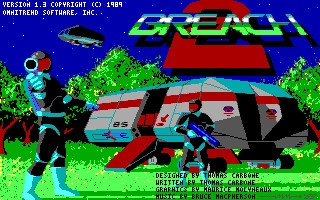This image captures a nostalgic screenshot from the retro video game "Breach 2," reminiscent of classic games from 20-30 years ago. The rectangular frame showcases a pixelated landscape with a vibrant blue sky and a verdant, green backdrop. Dominating the airspace is a sleek, black, futuristic craft flying mid-shot. The game's title, "Breach 2," prominently appears in the foreground on the right, with "Breach" in green and the numeral "2" in bold red.

On the ground below, another craft has landed, distinguished by its gray and red coloration and an extended ramp. Two spacemen in turquoise and black outfits, accented by red on their helmets, are present. One stands closer to the viewer, while the second figure appears more distant. The background is dotted with trees, featuring brown bark and lush green canopies, adding to the rich, immersive environment of the scene.